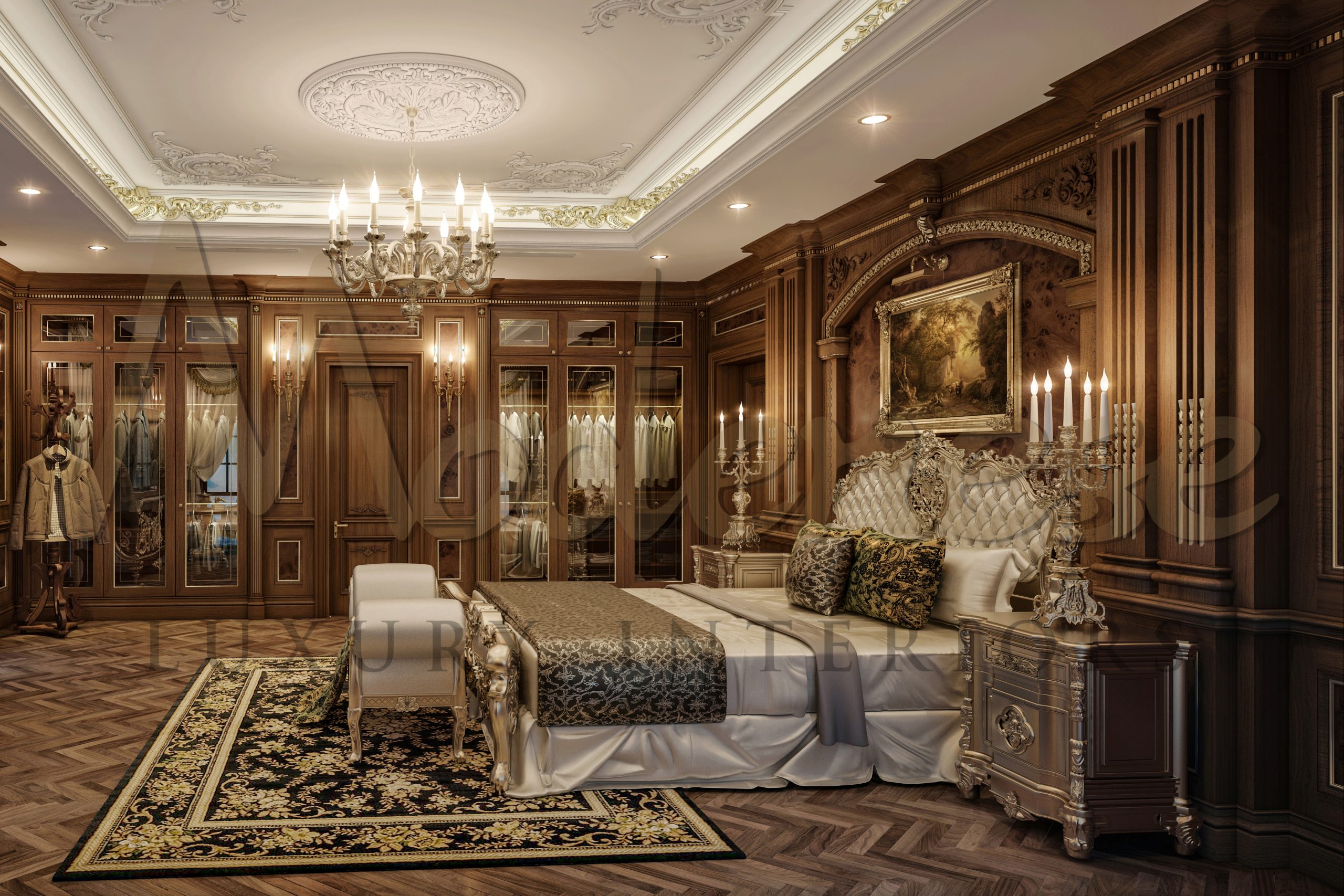This photograph captures an opulent bedroom designed for luxury and prominence. The room features exquisite wooden walls and trim, with the ceiling intricately detailed and adorned with gold accents around indented borders. A chandelier hangs in the center, providing an elegant focal point. Below, a plush bed is dressed in luxurious linens, including white satin sheets, gold and black leopard print pillows, and a matching blanket. At the foot of the bed, a Persian-style black and gold rug enhances the room's grandeur, while a white footstool with armrests stands nearby. Each side of the bed hosts an end table topped with candelabras, adding to the ornate ambiance. A clothes hanger mannequin with a jacket and a chandelier with many lights contribute to the sophisticated décor, completing this lavish interior setting.